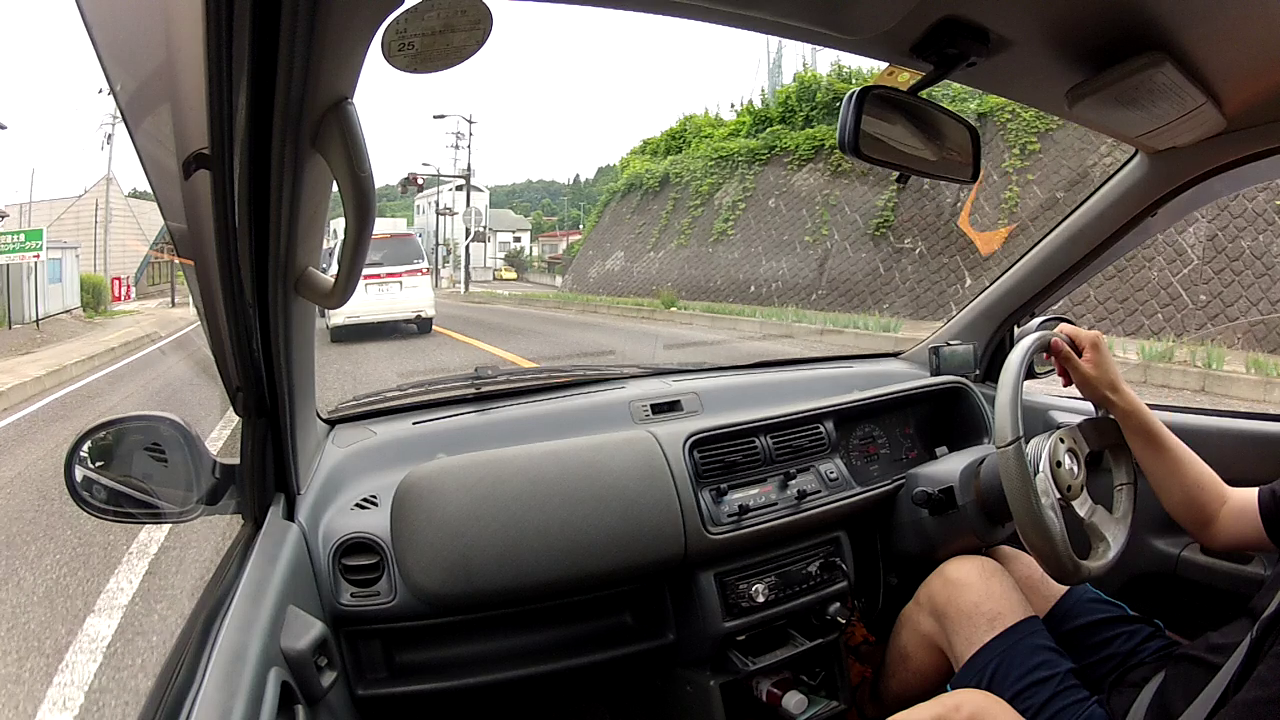This daytime photograph captures the view from the passenger seat of a right-hand drive car with a gray interior. Through the front and side windows, a clear street scene is visible. Directly ahead, a small white van occupies the lane, while the adjacent lane remains empty, emphasizing the two-lane road's spaciousness. On the right shoulder, a cement embankment adorned with lush greenery and cascading vines adds a touch of nature to the urban setting. To the left, buildings and a sidewalk line the road, contributing to the bustling environment. In the distance, streetlights punctuate the skyline, with more buildings and rolling hills providing a scenic backdrop.